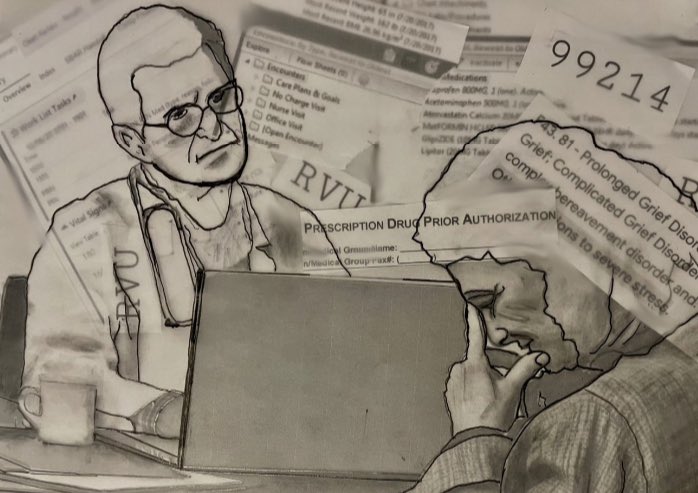The black-and-white line drawing depicts a somber interaction between two characters in what appears to be a medical or therapeutic setting. Seated at a desk, a doctor with a stethoscope is positioned behind an open laptop and a cup of coffee, gazing attentively at the person across from them. This second individual, presumably a woman, is visibly distressed, with her head bowed and a hand covering part of her face, conveying emotions of despair or frustration. The background features a chaotic collage of ripped paper bits and newspaper clippings, with notable fragments reading "Prescription Drug Prior Authorization," "Prolonged Grief Disorder," "Complicated Grief Disorder," and the code "99214." These elements hint at medical and psychological themes, possibly criticizing the bureaucratic complexities of modern healthcare. The scene is reminiscent of a comic illustration, utilizing sharp ink lines for a dramatic effect.